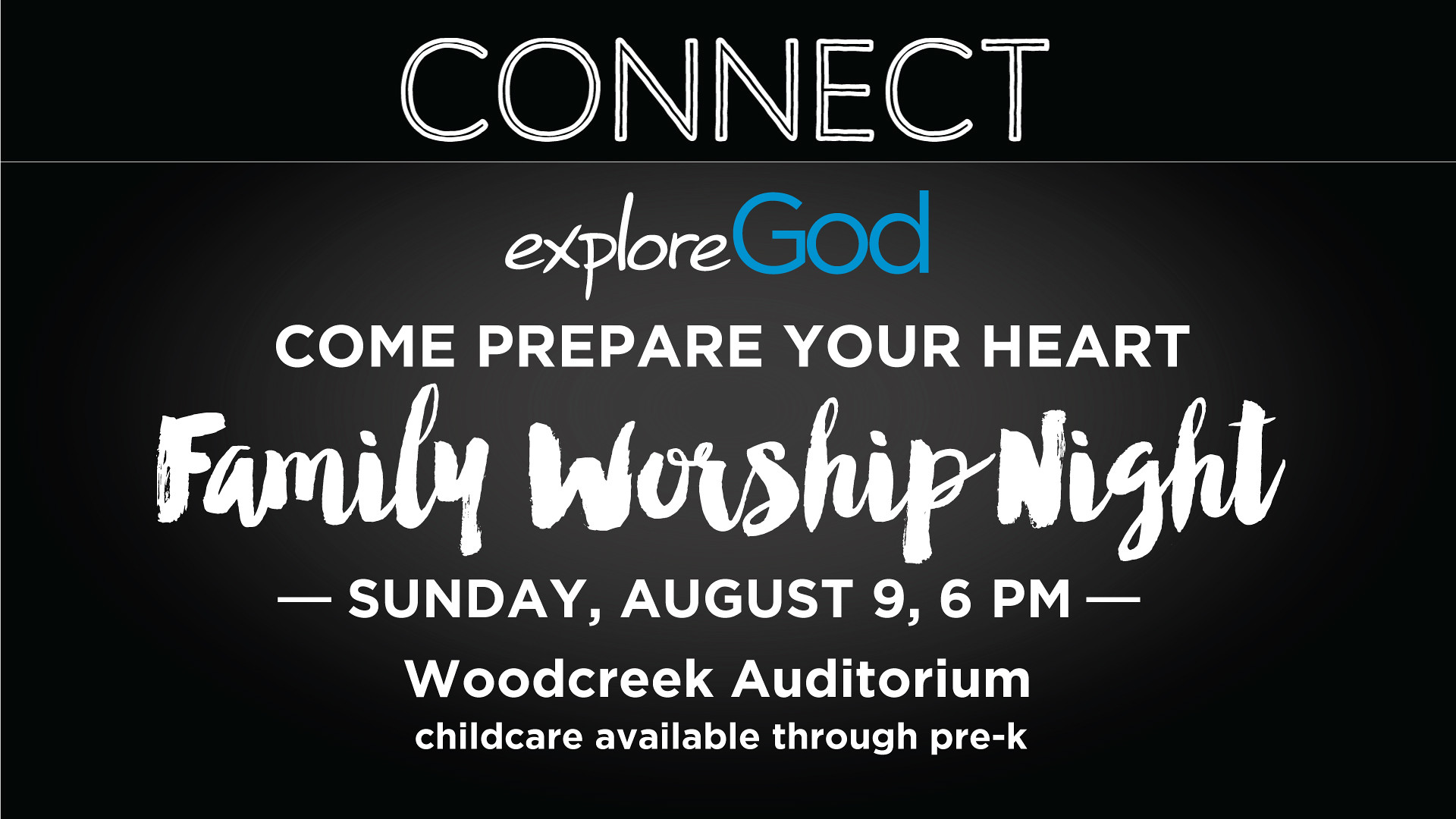The black poster features a solid black background with a faint grayish smudge in the center. Across the top eighth of the poster, a thin white line extends from left to right. Above this line, "CONNECT" is written in large, all-capital white letters. Below the line, the word "explore" appears in lowercase white letters, followed by "GOD" in uppercase blue letters. Underneath, another white line separates the next section with the phrase "COME PREPARE YOUR HEART" in all-capital white letters. In a bold cursive white font, the poster announces "FAMILY WORSHIP NIGHT". Below this, in all-capital white print, the details continue: "SUNDAY, AUGUST 9TH, 6PM" followed by another white line and then "WOOD CREEK AUDITORIUM, CHILD CARE AVAILABLE THROUGH PRE-K". Each line of text varies in font style, including block letters and cursive, to emphasize different parts of the message.